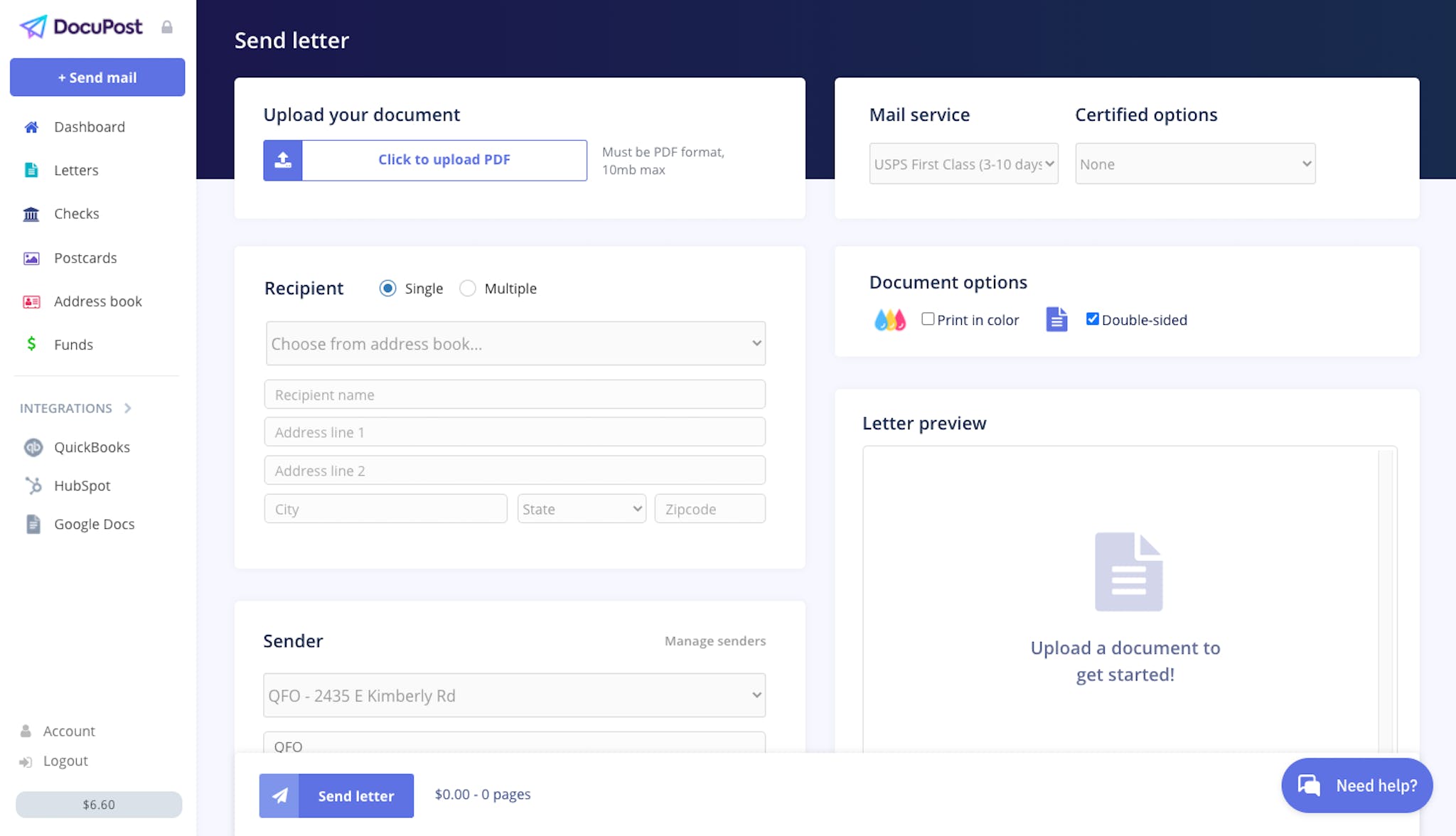A detailed screenshot of a webpage interface for 'DocuPost' is displayed. On the left-hand side, there is a vertical navigation column with 'DocuPost' at the top, accompanied by a logo of a paper airplane encased in a bluish-purple border. Directly below the logo is a prominent blue button labeled 'Send Mail.' Continuing down the column, several clickable options are listed: Dashboard, Letters, Checks, Postcards, Address Book, Funds, and Integrations, which include QuickBooks, HubSpot, and Google Docs. Near the bottom of the column, there are options for 'Account' and 'Logout.' Below these options, a gray total amount of $6.60 is displayed alongside a grayish button.

On the right-hand side of the screenshot, a navy-blue bar at the top features the text 'Send Letter.' Beneath this bar, there is a box labeled 'Upload Your Document,' with an upload button for users to submit a PDF file. The note specifies that the document must be in PDF format and no larger than 10 megabytes. Below this are fields to input information for the recipients, including options to specify between 'Single' or 'Married' status and a drop-down menu to choose from the Address Book. Additional input fields are provided for the recipient's name, address line one, address line two, city, state, and zip code.

Further down, there are sections for additional sender information. To the right, another drop-down menu labeled 'Mail Service' currently shows 'USPS First Class, 3 to 10 days' as the selected option, with 'Certified Options' set to 'None.' Below this, under 'Document Options,' there is a checkbox for 'Printed Color,' which is not checked, and another for 'Double-Sided,' which is checked. At the bottom, there is a 'Letter Preview' box providing a visual representation of the letter to be sent.